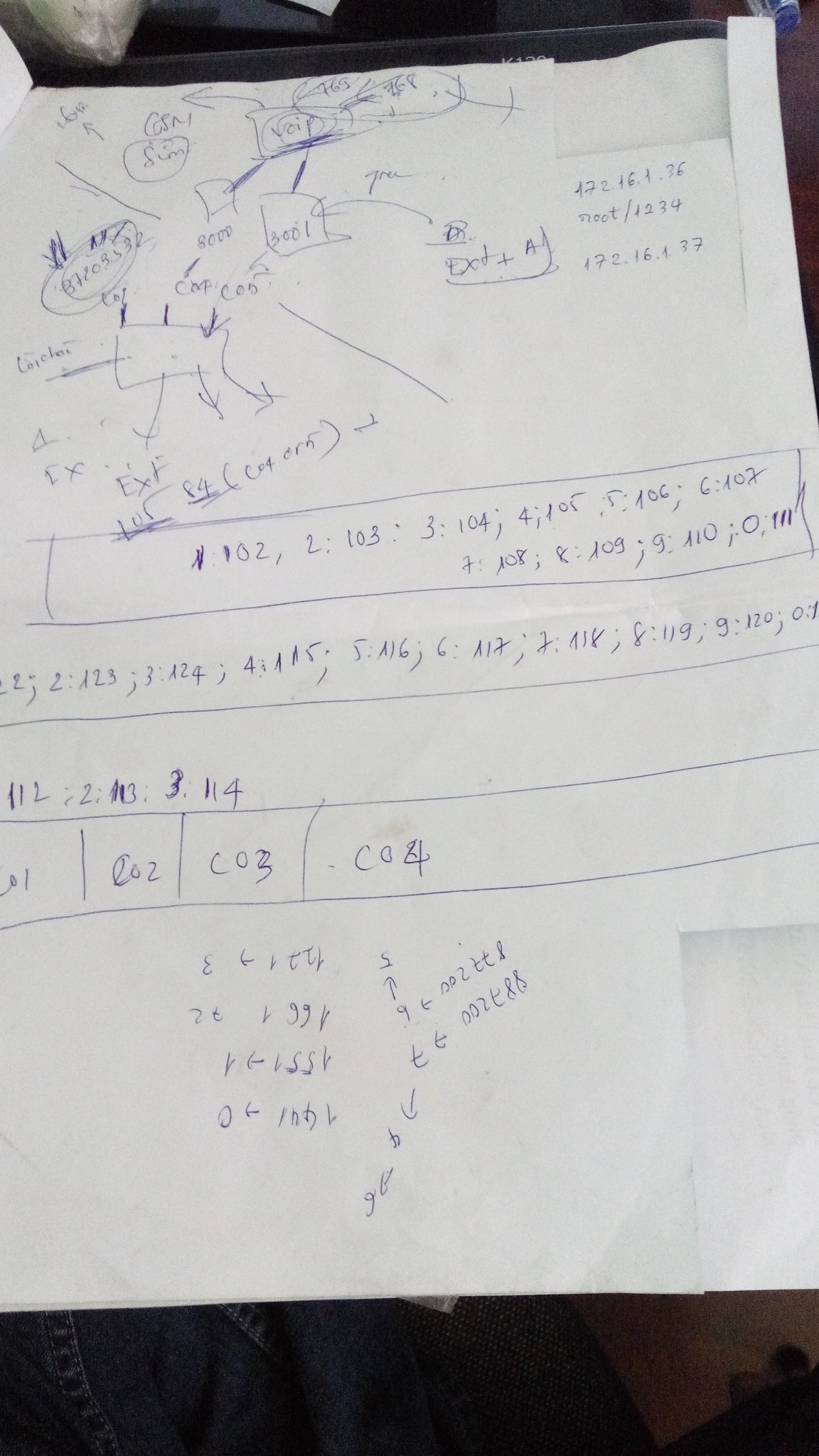The image captures a close-up of a piece of blue paper filled with handwritten notes. At the top of the page, hastily jotted scribbles dominate the space, featuring a mix of circles, squares, numbers, letters, and arrows pointing in various directions. The annotations are cryptic and lack context, making it difficult to decipher their exact meaning.

To the right of the scribbles, a sequence of numbers and symbols is neatly written:
- 17216.1.36
- root/1234
- 17216.137

Below this sequence, a horizontal box spans the width of the paper, filled with a structured series of numbers separated by colons and semi-colons. The entries read as follows:
- 102,2:103:3:104;4:105;5:106;6:107
- 7:108;8:109;9:110;0;111

Below these entries, the pattern continues with more numbers and letters organized in a similar fashion. The rest of the paper contains more lines drawn horizontally, each interspersed with additional numerical and alphabetical annotations. Overall, the notes appear complex and seem to follow a specific, albeit unclear, schema only understandable to the note-taker.